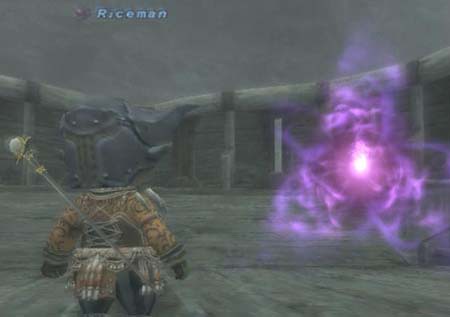A scene from a movie depicts a mysterious figure donning traditional samurai-like armor, characterized by protective, non-metallic gear. Positioned left-center, the frame features the title "Riceman" written in white font near the top. The overall color palette of the image is dominated by grayish tones. The enigmatic armored figure, adorned with a large helmet or headgear, is intently facing an ethereal, purple-hued being on the right side of the frame. A visible weapon extends from behind the samurai-like character, suggesting a sense of readiness or conflict. The scene evokes a fantastical atmosphere, hinting at a storyline suitable for children.